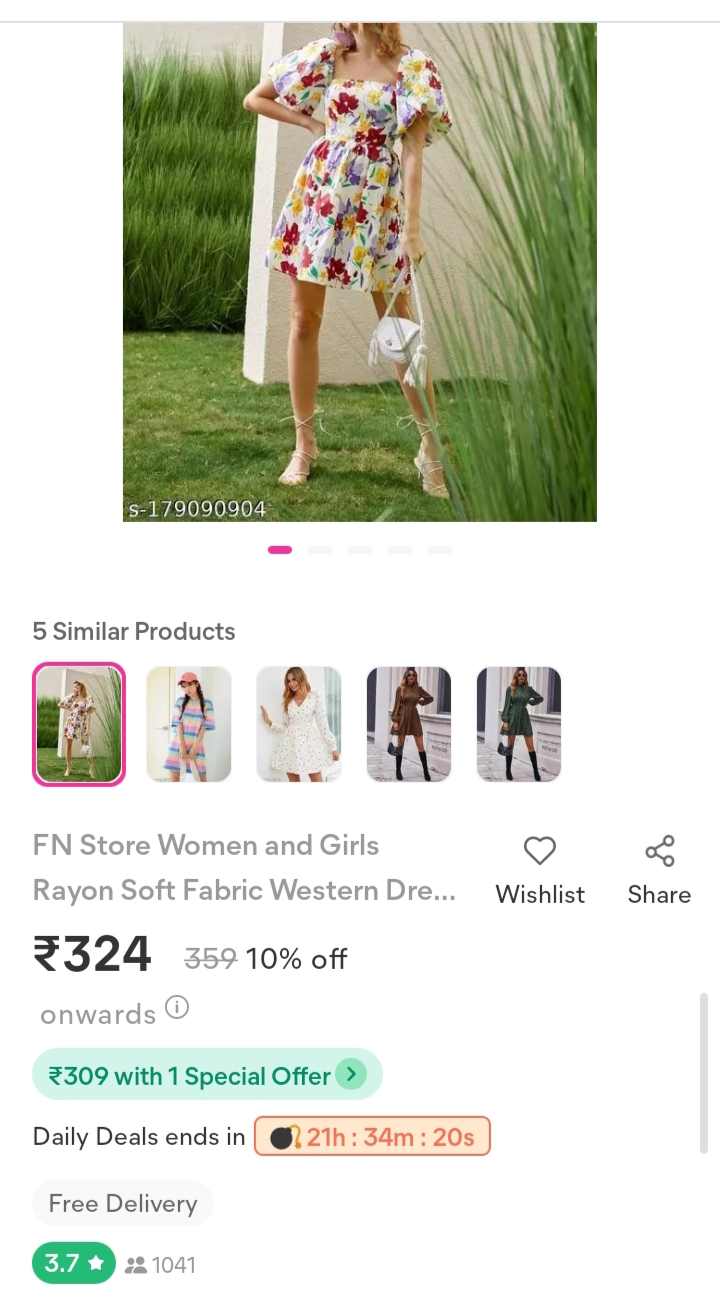A zoomed-in image from an unspecified shopping website displays a woman from her shoulders down, set against a background that features green grass on the left and a white wall on the right. She is dressed in a vibrant floral dress adorned with white, purple, yellow, and red flowers. Complementing her dress, she carries a white pocketbook and wears strappy sandals.

The bottom left corner of the image contains text in white: "s1790909094," and below this in black, it says: "Five Similar Products." Displayed underneath are four thumbnails of other dresses including the current one, which is highlighted with a magenta outline. The first dress features various shades of purple, yellow, and green, the second dress is white, and the third is brown. Another thumbnail shows the same dress in green.

In gray text, the website lists: "FN Store Women and Girls Fine On Soft Fabric West Dress" priced at an unknown currency 324 with a 10% off discount. Additional text mentions "Daily Deals" and a countdown timer, indicating "21 hours, 34 minutes, 20 seconds" remaining for free delivery.